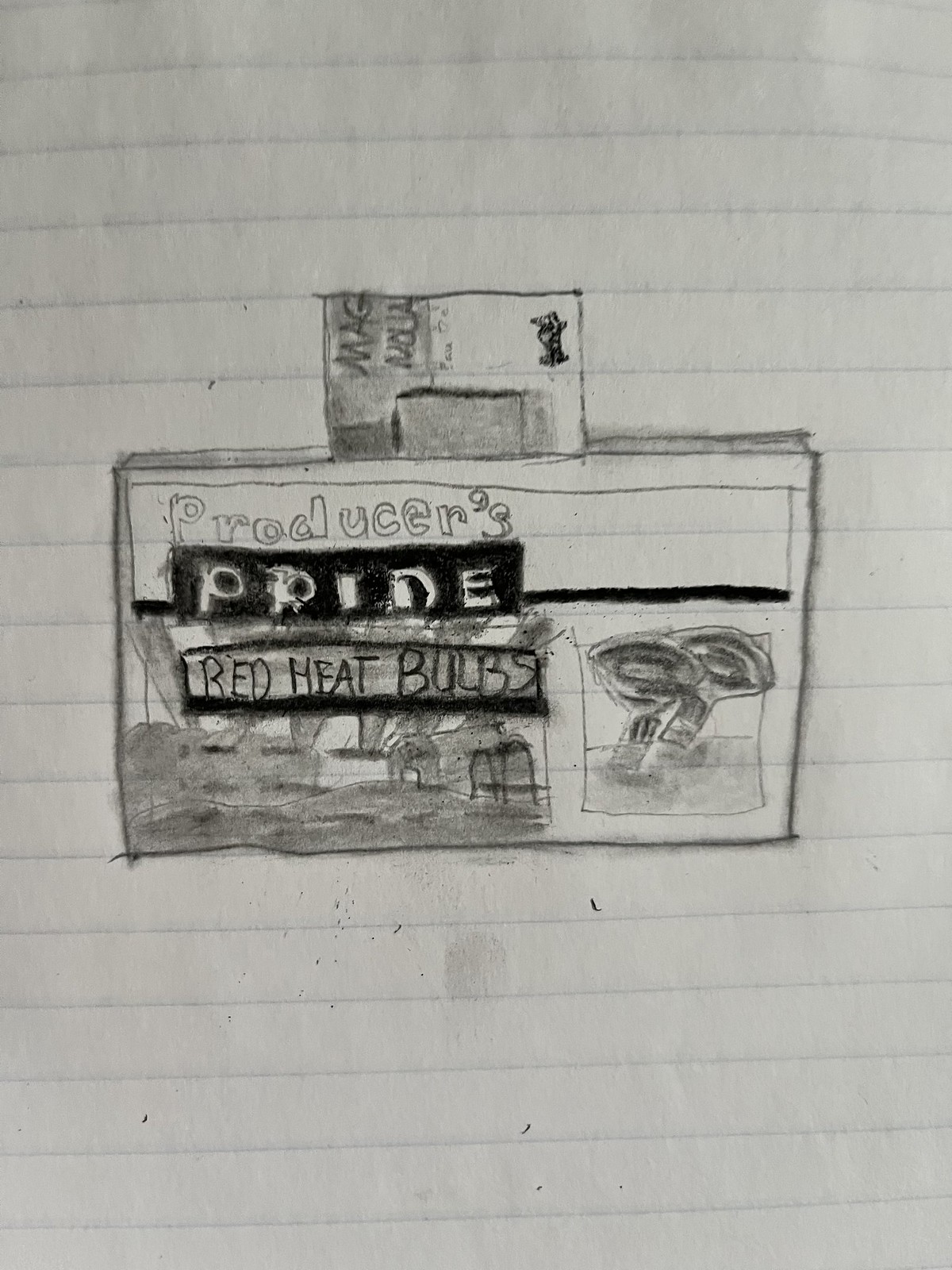The photograph, in portrait format and in color, zooms in on a piece of lined notebook paper serving as the canvas for a somewhat rough pencil sketch. The sketch depicts a rectangular box, possibly a container for light bulbs, with notable labels and imagery. Dominantly positioned across the front of the box are the words "Producers Pride" outlined in a dark, shaded rectangle, and below it, "Red Heat Bulbs." The drawing includes uneven depictions of two light bulbs alongside the text, reinforcing its purpose. Additional details suggest impressions of letters, likely from prior writing on the preceding page, subtly imprinted on the paper. There is a handle on the top of the box, rendering it as an imperfect yet recognizable image of a light bulb package.